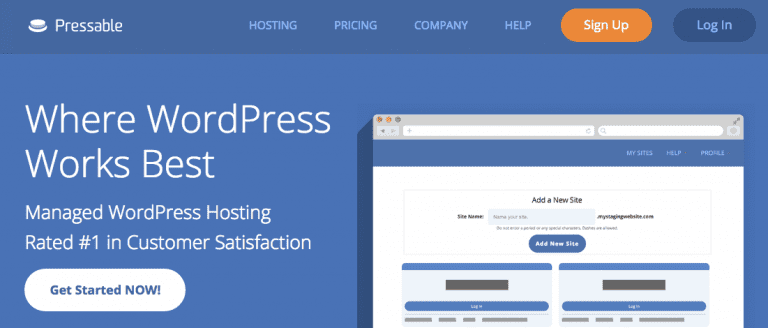This web page features a predominantly blue background and a horizontally elongated rectangular layout. The top left corner prominently displays the "Pressable" logo. To the right, there is a horizontal navigation menu including the following options: "Hosting," "Pricing," "Company," and "Help," followed by an inviting "Sign Up" button presented in an orange box with white text. In the top right corner, a dark blue box contains a "Log In" link in lighter blue text.

On the left side of the page, the slogan "Where WordPress Works Best" is showcased as the largest text on the page, conveying a clear and bold message. Beneath this, a subheading states, "Managed WordPress Hosting. Rated number one in customer satisfaction," highlighting the service's accolades. Below this subheading, a white box with blue text invites users to "Get Started Now."

To the right side of the page, there is an illustrated depiction of a website interface with a gray-bordered header. The text within the image reads "My Site's Help Profile," followed by an "Add a New Site" option. It includes a "Site Name" field with a rectangular input box for entering information. Below this input box, there is some blurry text that is difficult to discern but possibly says "Log In."

This detailed description encapsulates the visual elements and textual content of the web page, emphasizing both its functional and aesthetic qualities.